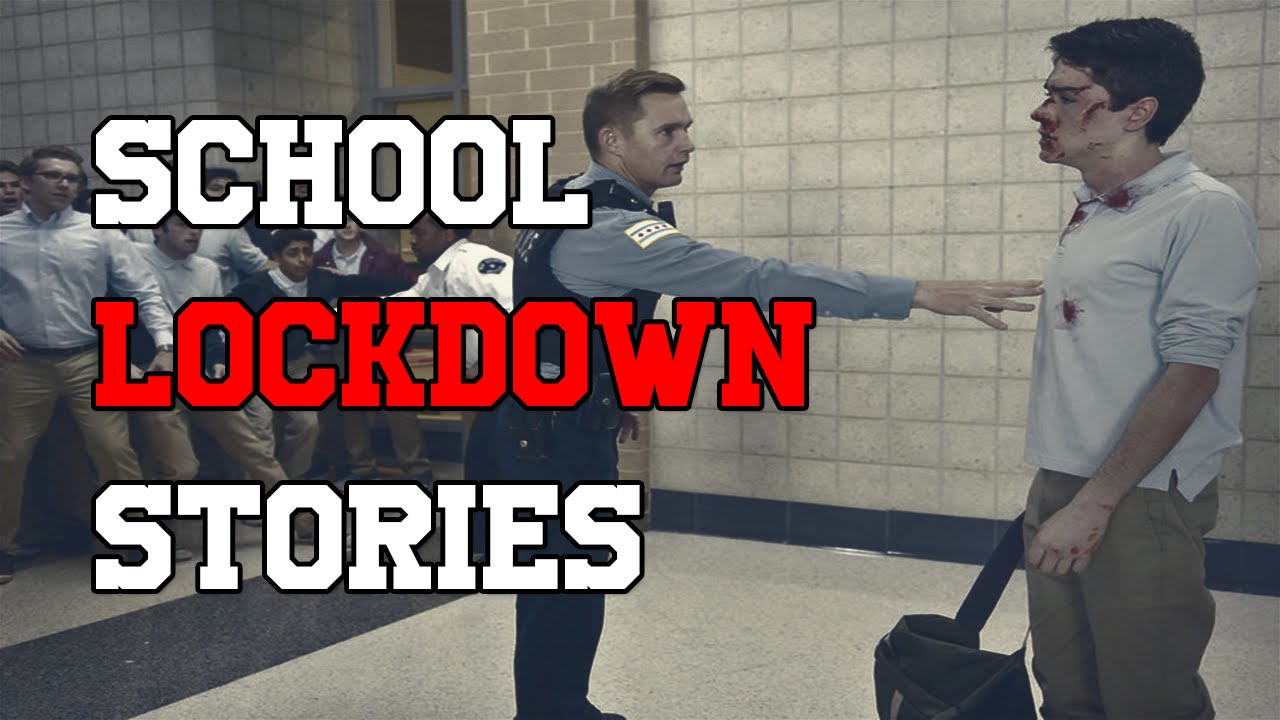The image captures a tense scene featuring a police officer and an injured student amidst what appears to be a school conflict. The police officer, dressed in a light blue long-sleeved collared shirt, a police vest, and dark pants, extends his hand toward the chest of the student, who has blood on his face and white long-sleeved collared shirt rolled up to his elbows. The student, who is fair-skinned with short dark hair, is wearing khaki pants and holding a black bag slumped to the floor. Blood is evident on his shirt and face.

Behind the police officer, a second officer in a white shirt with a badge is holding back a crowd of students, some appearing to be in a fight stance. The background features white tiled walls and some brickwork. Prominently displayed across the image are the words "SCHOOL LOCKDOWN STORIES" in all caps, with "school" and "stories" in white and "lockdown" in red. The atmosphere is charged with tension, highlighted by the positioning and expressions of the individuals present.